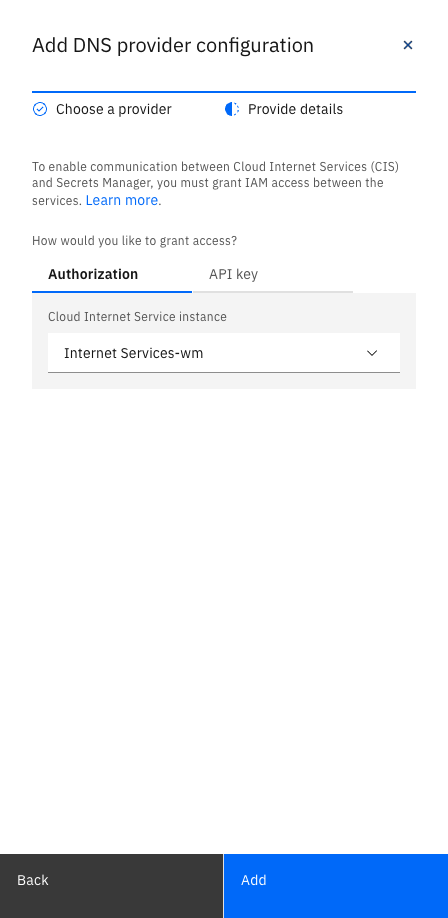At the top of the image, there is a header with the text "ADD DNS Provider Configuration," all in capital letters and in black font. To the right of this header, there is a small "x" icon. The header is underlined with a dark blue horizontal line. 

Below the header, there is a section titled "Choose a Provider," featuring a blue checkmark inside a blue-outlined circle. To the right of this section, half of the circle is blue and the other half is white, with the text "Provide Details" in black font. 

The subsequent text reads: "To enable communication between Cloud Internet Services (CIS) and Secrets Manager, you must grant IAM access between the services." Below this, there is a blue underlined link labeled "Learn More."

The next prompt asks, "How would you like to grant access?" followed by the text "Authorization" in black font, which is also underlined in blue, and to the right, the option "API Key" in gray font.

Underneath this, there is a field labeled "Cloud Internet Service Instance" with a long input box below it, containing the text "Internet Services - WM."

At the very bottom of the image, there are two buttons: a dark gray box on the left with the word "BACK" in white font and a blue box on the right with the word "ADD" also in white font.